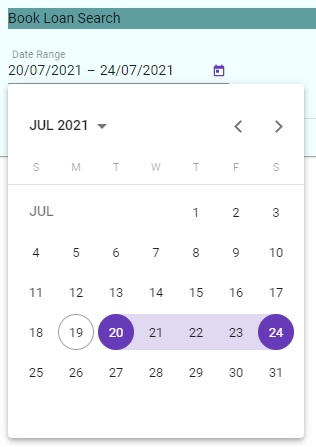The image showcases an interface for a book loan search tool, featuring a green box labeled "Book Loan Search" at the top. Below this, there is a light green background containing the text "Date Range: 20-7-2021 to 24-7-2021." Displayed prominently is a calendar for the month of July 2021. On the right-hand side of the calendar, there are navigational arrows allowing users to move between different months. Key dates are highlighted; the 19th is encircled in gray, the 20th and 24th are circled in purple, and the days between the 21st and 23rd are marked with a lavender background.